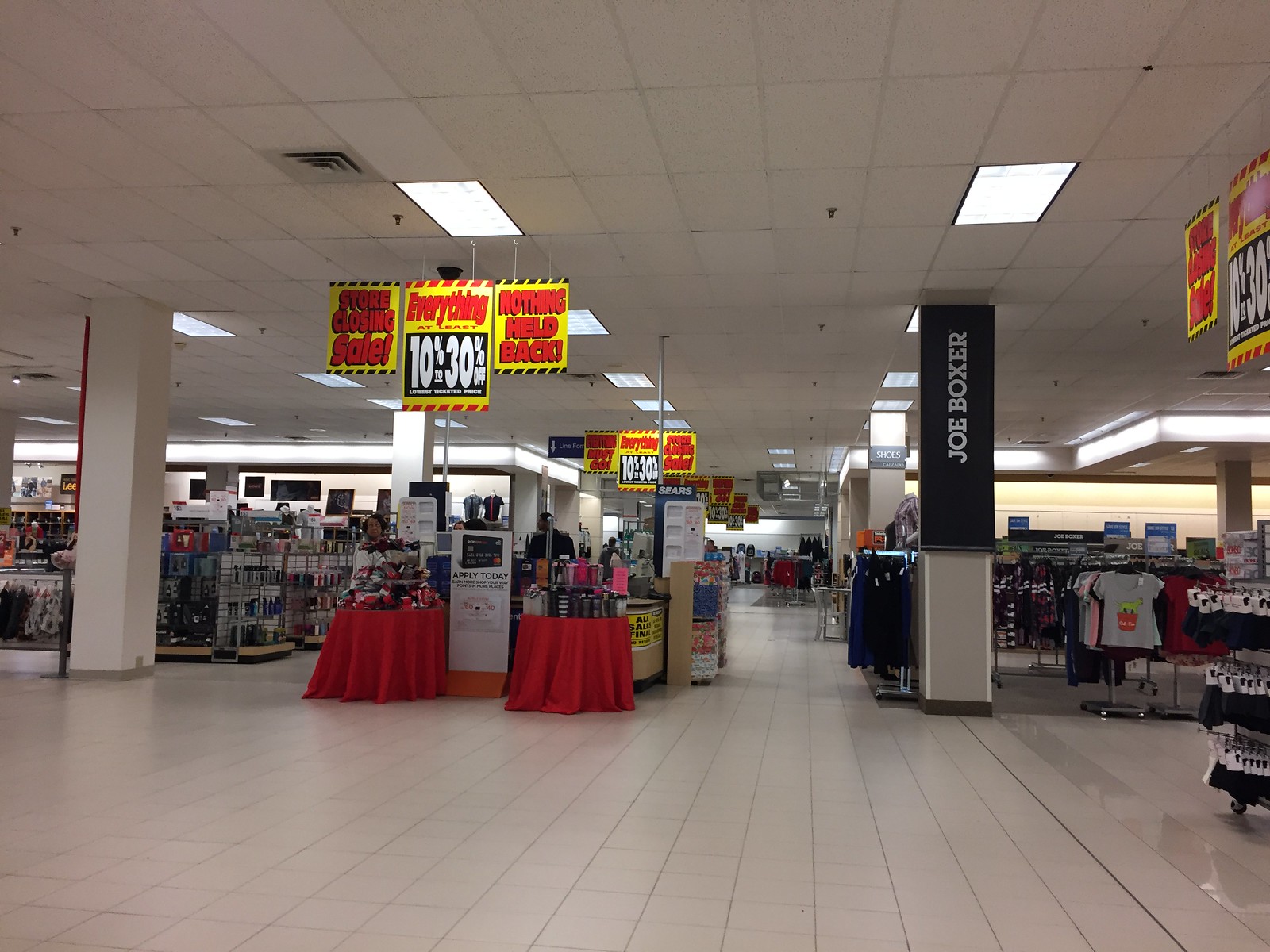The image depicts the interior of a store having a clearance sale. The floor is covered with white square tiles, delineated by black lines that form a grid pattern. Prominently displayed overhead is a series of signs hanging from the ceiling. The leftmost sign is a yellow rectangle with black dashed borders and features bold red text that reads "Store Closing Sale." Adjacent to this sign, also in red text on a similar yellow and black background, are the words "Everything at Least." The sign continues with "10% to 30% Off Lowest Ticketed Price" in white text. Completing the series, a sign declares "Nothing Held Back" in red font atop a yellow and black backdrop.

On the right side of the image, there is a display of children's short-sleeve clothing, including one item featuring a graphic of a cat. Nearby, a prominent black sign with white text reads "Joe Boxer," indicating the brand of the clothing.